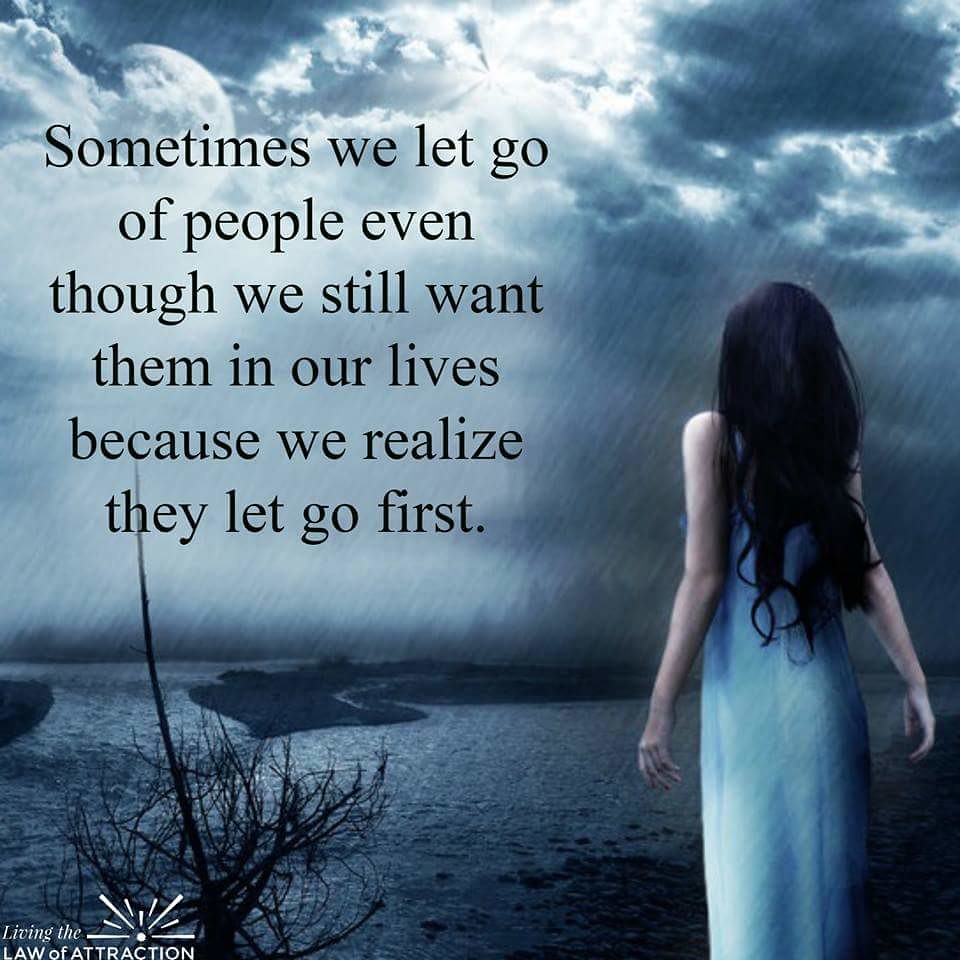A young woman stands on the right side of a stormy beach scene, her long black hair cascading down to her waist. Clad in a flowing, light blue gown tinted darker by the gloomy lighting, she extends her arms slightly outward. She faces the dark, calm waters beneath an ominous, rain-laden sky, with beams of sunlight attempting to break through the dense clouds above. Sparse beach grass and a small, sandy island are visible near the bottom of the image. On the left side, six lines of black text read: "Sometimes we let go of people even though we still want them in our lives because we realize they let go first." The lower left corner features a circular symbol with radiating lines, associated with the concept of 'Living the Law of Attraction.'